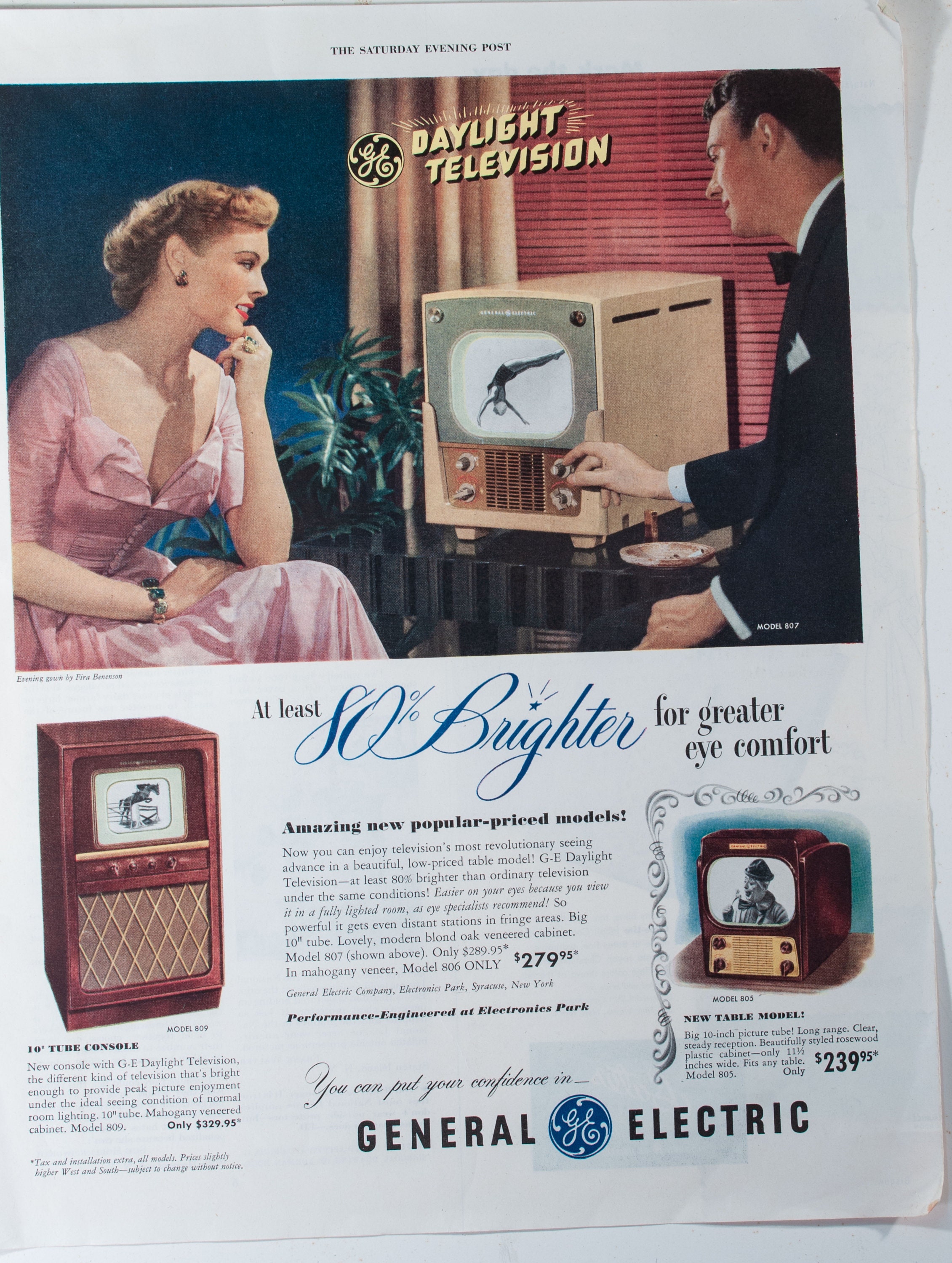This is a full-page vintage advertisement from the late 1940s or early 1950s for General Electric, featured in the Saturday Evening Post. The ad showcases GE's "Daylight Television" with a colorized, animated illustration occupying the top half of the page, depicting a man and woman enjoying an early television set. The TV is prominently large and cubical with a small, rounded square screen at the top and four knobs below a large audio grill. The television appears to show a diver mid-air on the screen. Both individuals are seated in a stylish living room with blue walls, brown curtains, red window frames, and an array of indoor plants.

The woman is elegantly dressed in a pink gown with blonde hair, accessorized with earrings and a green wristband, while the man, with black hair, is outfitted in a black suit and a white shirt. Below this scene is a footnote crediting the evening gown to designer Eva Bernon.

The bottom half of the ad emphasizes the tagline "At least 80% brighter for greater eye comfort" in large, creative blue font. The ad also presents two alternative GE television models on the left and the right sides of the page. The model 809, priced at $329.95, features a mahogany veneer and a 10-inch tube. On the central part of the page, it highlights the benefits of the new GE Daylight Television, which is at least 80% brighter than ordinary TVs and more comfortable for the eyes in a fully lit room. The model 807, in blonde oak veneer, is available for $289.95, and the model 806, in mahogany veneer, at $279.95. Another model, the 805, is displayed on the right, showcasing a compact, beautifully styled rosewood plastic cabinet, and is priced at $239.95.

At the bottom of the ad, the General Electric name and logo are prominently displayed with the tagline, "You can put your confidence in General Electric."